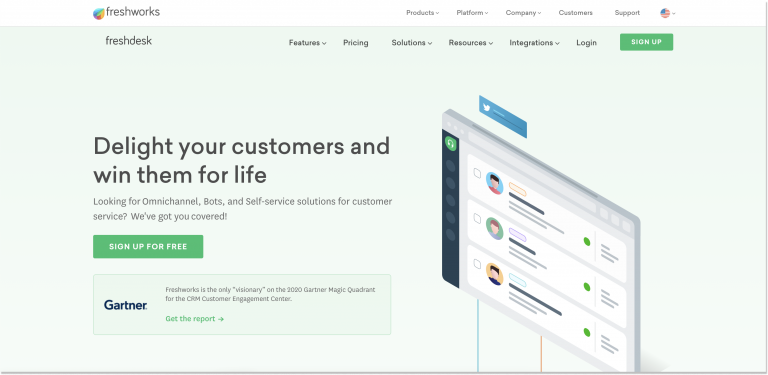This is a detailed screenshot of a webpage taken from a laptop screen, which is landscape in orientation, approximately twice as wide as it is tall, and surrounded by a gray border along the right edge and bottom. 

At the very top of the screenshot, there is a white rectangular page header with the word "Freshworks" in gray font, along with a colorful, rainbow-like spherical logo positioned centrally on the left side. To the right of this logo, several dropdown menu options are displayed in gray font, including "Products," "Platform," and "Company." Additionally, there are clickable buttons labeled "Customers," "Support," and a language selector featuring an American flag enclosed in a circular icon.

Below the main header, a green rectangular border reads "Freshdesk" and features submenu options across the top, including "Features," "Pricing," "Solutions," "Resources," "Integrations," and "Login." A green "Sign Up" button with white font is also visible within this section.

The primary headline on the page reads "Delight your customers and win them for life," positioned above another green, rectangular sign-up box with white font that says "Sign Up for Free." Below this call-to-action, the word "Gartner" appears, suggesting a related topic or endorsement.

To the right side of the screenshot, an image of a computer screen is visible, complementing the textual content on the left.